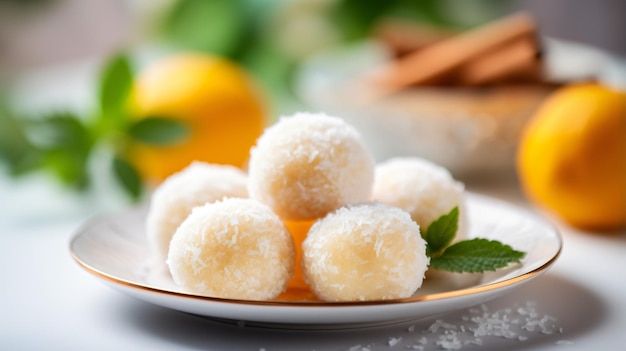This photograph features a close-up, top-down view of a white, circular plate with a delicate gold rim, which holds five round cookies. The cookies have a light yellow hue and are generously coated with fine white granules of sugar. Four cookies are arranged on the plate, with the fifth cookie artistically stacked on top of the others at the center. To the right and slightly below the plate, a small pile of scattered sugar granules can be seen, adding to the rustic charm of the presentation.

The background of the image is soft and muted, drawing focus to the plate and its contents. On the right side of the composition, a vibrant lemon is placed next to a white bowl containing aromatic brown cinnamon sticks. Adjacent to these elements, there's an orange, partially visible, with a few green leaves adding a touch of color, despite being out of focus. Additionally, two fresh basil leaves protrude from the right side of the cookies, enhancing the overall visual appeal and providing a hint of freshness. This arrangement creates a harmonious blend of textures and colors that amplify the allure of the cookies.